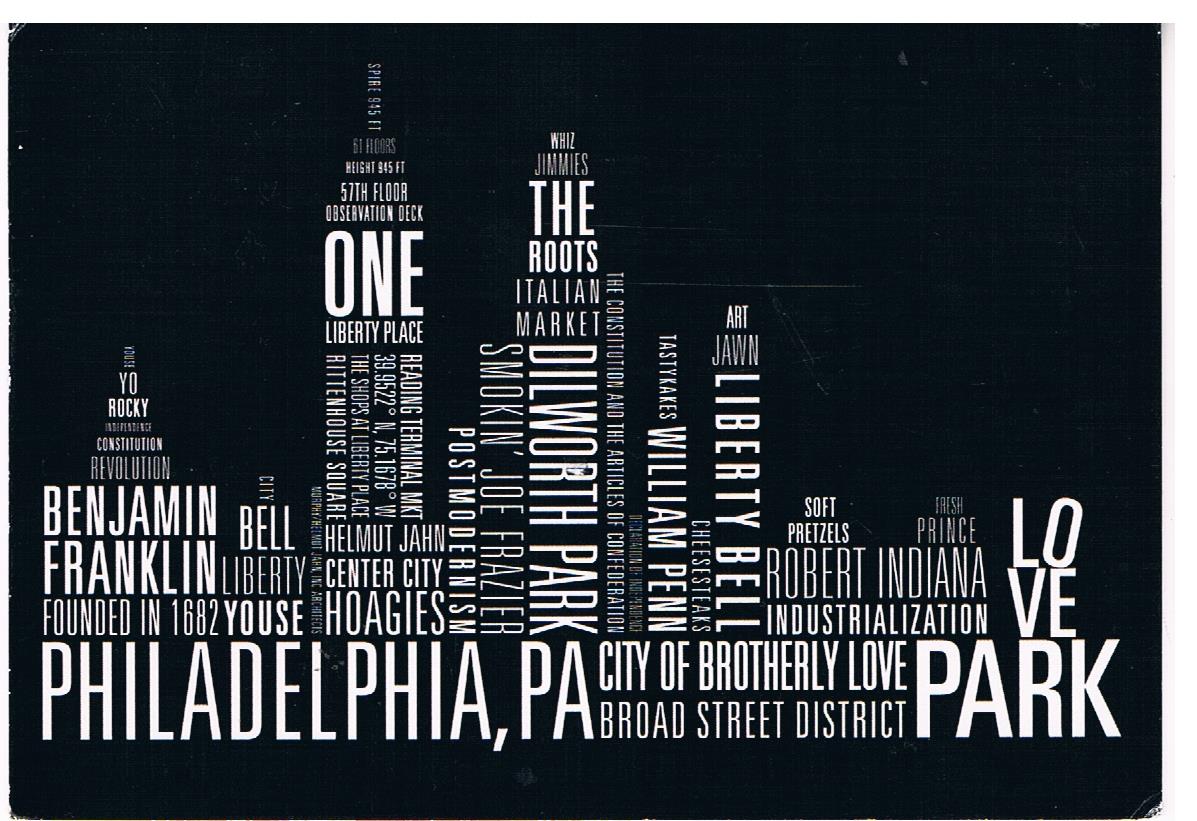The image features an artistic poster with a black background and white text forming the skyline silhouette of Philadelphia. At the bottom, in prominent lettering, it reads "Philadelphia, PA, City of Brotherly Love, Broad Street District, Park." Above this, various words and phrases associated with Philadelphia are arranged in different fonts and sizes to mimic the architecture of buildings. These include terms like “Yo Rocky,” “Constitution Revolution,” “Benjamin Franklin,” “Liberty Bell,” “One Liberty Place,” “Helmut John,” “Center City Hoagies,” “The Roots,” “Italian Market,” “Dilworth Park,” “William Penn,” “Love,” “Soft Pretzels,” “Fresh Prince,” “Robert Indiana Industrialization,” and “Love Park.” The creative typography encapsulates the essence and iconic elements of Philadelphia, blending historical references with cultural landmarks, all meticulously structured to depict the city’s skyline in text form.